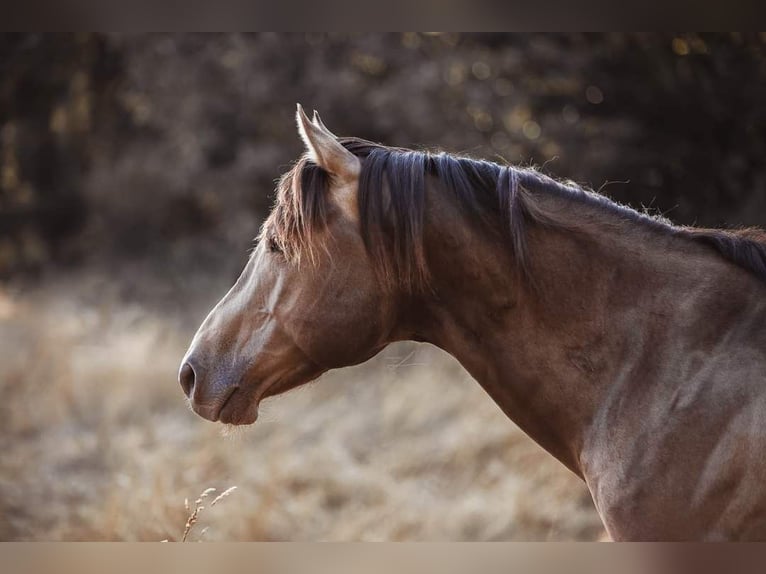The photograph captures a detailed side profile of a brown horse, positioned with its head and neck in sharp focus and looking intently to the left. The horse's coat is a pretty, light brown hue, and its mane is styled with part draped over the left side and the rest cascading to the right. The horse's forelock is visible between its attentive ears, which are pointed forward. The muscular build of its shoulder and outstretched neck emphasize its strong physique. Its black mane extends from the top of its head, down the back of its neck, to the upper part of its body. The picture cuts off at the shoulders, leaving the rest of the body blurred into the background. The background is a blurred mix of trees and dried, sun-bleached grass, indicating a late afternoon setting, casting natural light over the scene. The horse's focused gaze and flared nostrils suggest it is observing something interesting off-frame. The overall composition directs attention solely to the horse, with its surroundings soft and indistinct.